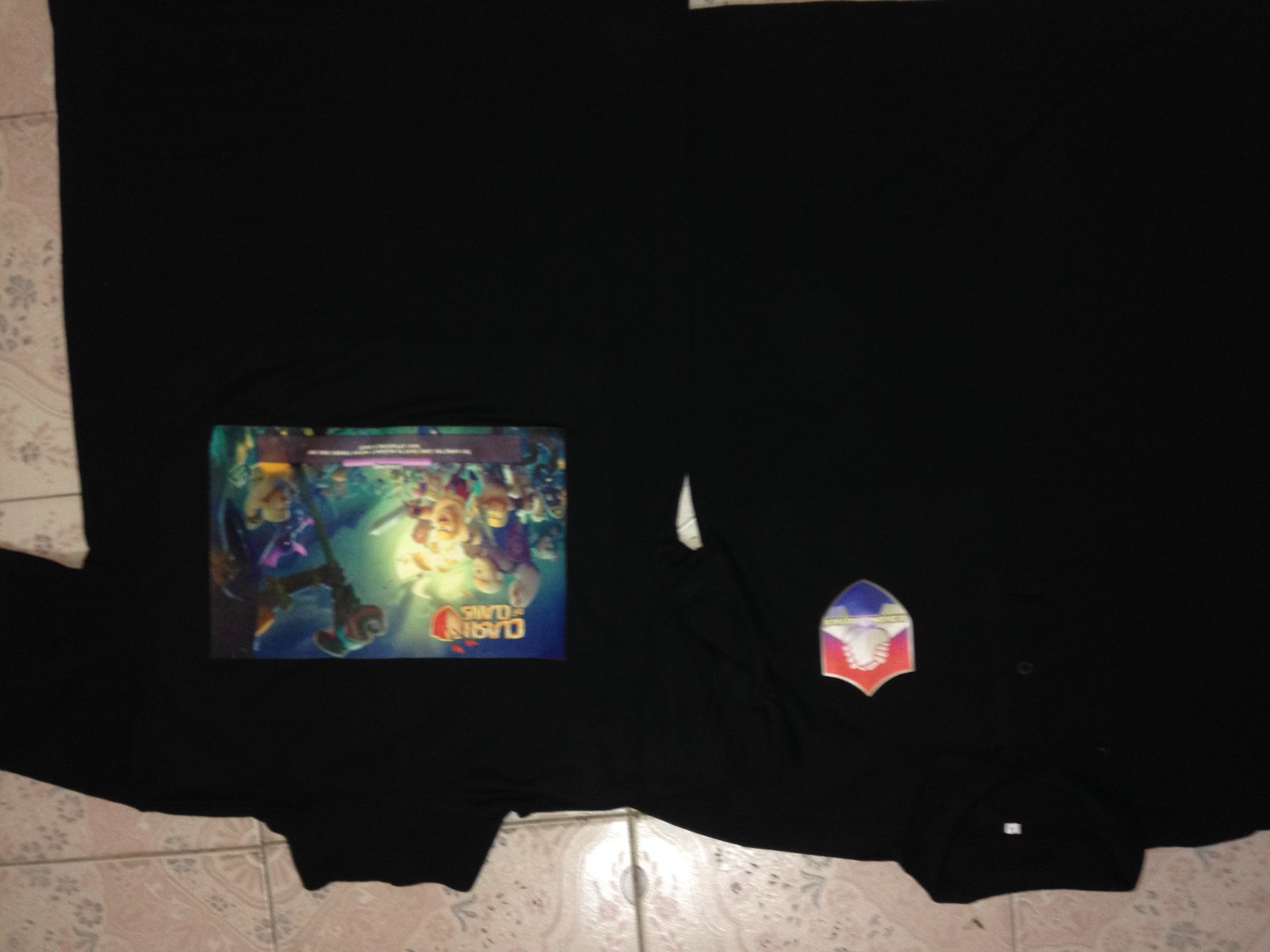The image consists of two sections, showcasing a shirt laid flat on a tiled floor with a distinct pattern. The left side presents the front view of the shirt, while the right side exhibits the back view. 

The back of the shirt features a prominent print of a loading splash screen from the popular mobile game Clash of Clans, depicting an intense scene with warriors engaging in combat. 

Meanwhile, the front of the shirt is adorned with a pocket on the left side, which carries an upside-down shield emblem. The shield design is colored with red at the top and sides, blue at the bottom, and features two hands clasping each other in the center.

This descriptive caption provides a detailed visualization of the shirt's design elements and the overall layout of the image.